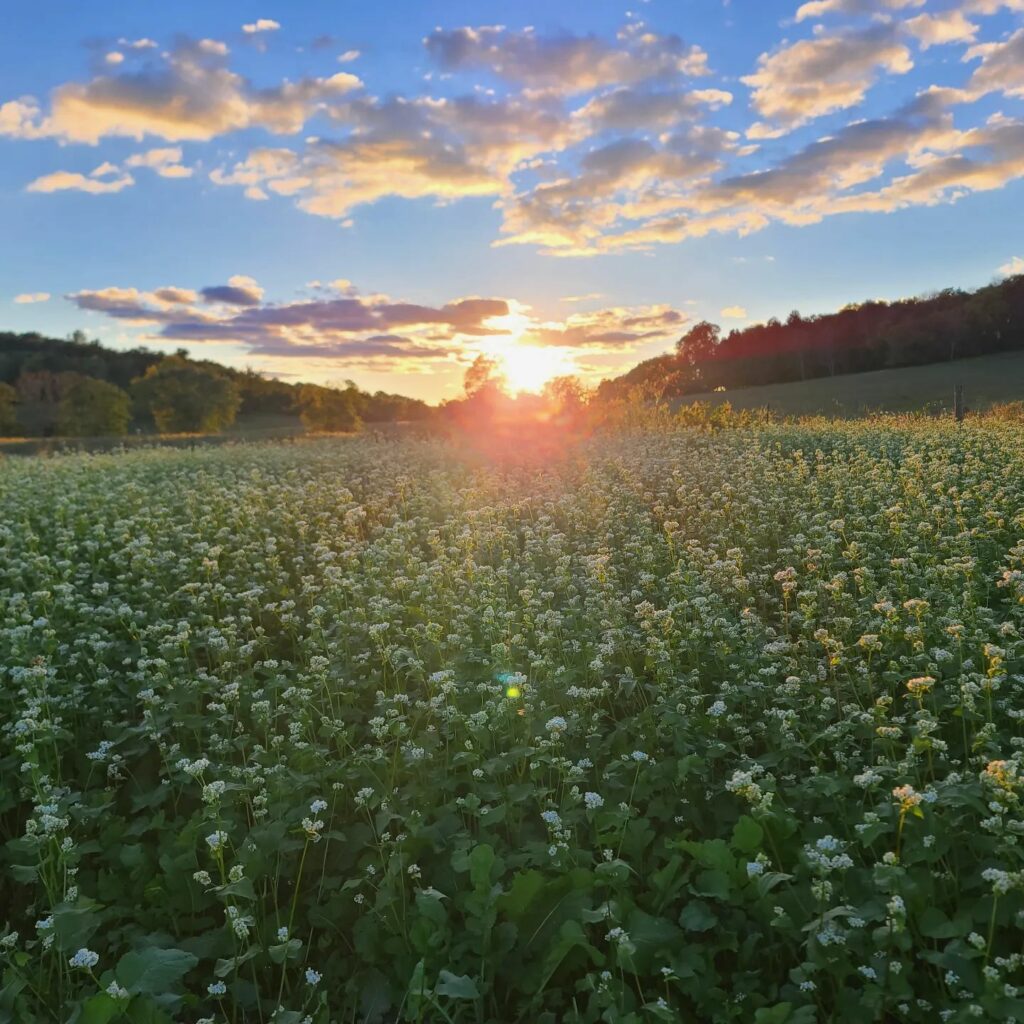The vertical photograph captures a serene landscape just as the sun sets, casting a golden hue over the scene. In the foreground, a lush field is teeming with tall green plants adorned with white flowers. The perspective narrows dramatically as the field stretches into the distance, leading the viewer’s eye toward the horizon. On either side of the field, grassy hills rise gently, dotted with trees. Above, the sky shifts from a deepening blue to a palette of gold and orange around the edges, where the sun is just slipping below the horizon. Scattered white and gray clouds also reflect these warm tones, creating a harmonious blend of colors that emphasizes the tranquility of the moment. The overall setting suggests a calm, clear evening with no indication of impending weather changes.